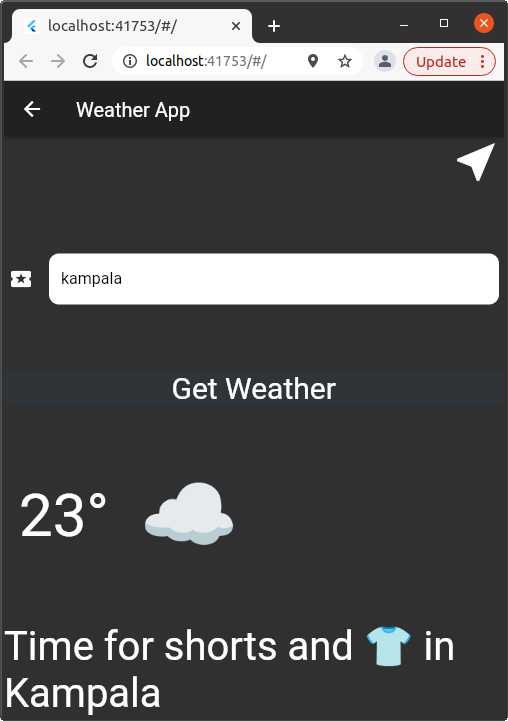A detailed look at a smartphone screenshot reveals a local host webpage displayed in a browser, lacking visible elements like the top bar that shows time and battery life. The URL bar, set to "localhost" with a specific port number, features buttons for refreshing the page, pinning the tab, marking it as important, and managing your account. A triplet of dots allows for additional settings. Below, the content reveals navigation buttons with one indicating the current weather application. Enter Kampala in the search bar to generate results on a sleek black background. Central, white text reads "Get Weather," and beneath this, the display shows it is 23 degrees Celsius and cloudy, with a message: "Time for shorts and t-shirts in Kampala," confirming the use of centigrade for temperature.